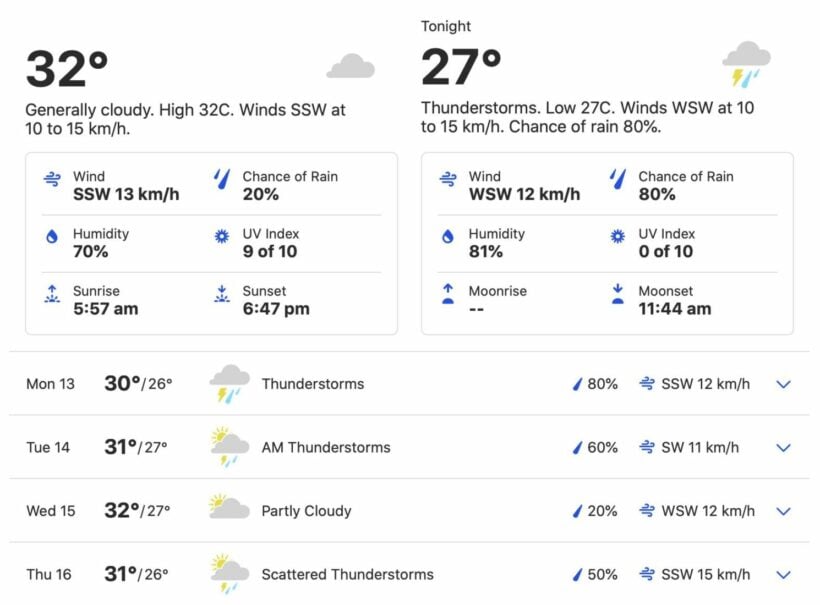The image displays a weather forecast webpage, divided into neatly organized blocks of information, each containing crucial weather details for the viewer. 

On the left side, the first block indicates the daytime forecast: 
- Temperature: 32°C
- General Weather: Mostly cloudy
- High: 32°C
- Wind: Southerly, specifically SSW, blowing at 10-15 mph 
Additional indicators include wind speed, humidity levels, sunrise and sunset times, UV index, and chance of rain.

Adjacent to it on the right is the nighttime forecast: 
- Temperature: 27°C
- General Weather: Thunderstorms 
- Low: 27°C
- Wind: Westerly, WSW, blowing at 10-15 mph
- Chance of Rain: 80%
This block is visually enhanced with a rain cloud icon, complete with lightning and raindrops. Additional details provided in this block include wind speeds, humidity, moonrise times, chance of rain, UV index, and sunset times.

Beneath these primary blocks, it outlines the forecast for the upcoming days—Monday through Thursday (the 13th to the 16th). Each day shows the weather conditions with appropriate symbols, such as clouds and thunderstorms, and details the type of weather expected (e.g., partly cloudy, scattered thunderstorms), percentage chance of precipitation, and wind direction.